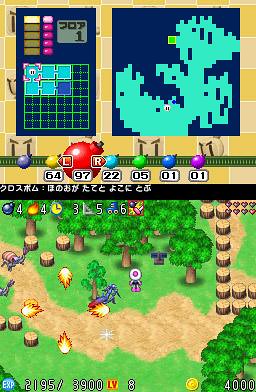This image is a screenshot from a video game and is separated into two distinct parts, akin to the dual screens of a DS Lite. The top screen features a pixel art illustration of a duck, set against a dark blue square background. The depiction is composed of turquoise squares that form a rough, simplistic shape of a duck. On the left side of this screen, there is a grid containing squares filled with either blue or turquoise colors. Japanese characters are displayed at the top of this section.

The bottom screen presents a 2D/3D top-down view of a character navigating through a landscape dotted with various elements. A defined pathway winds through the terrain, which is bordered by logs that function as a makeshift fence. The environment is populated with trees, including a mix of fully grown trees and stumps from trees that have been cut down.